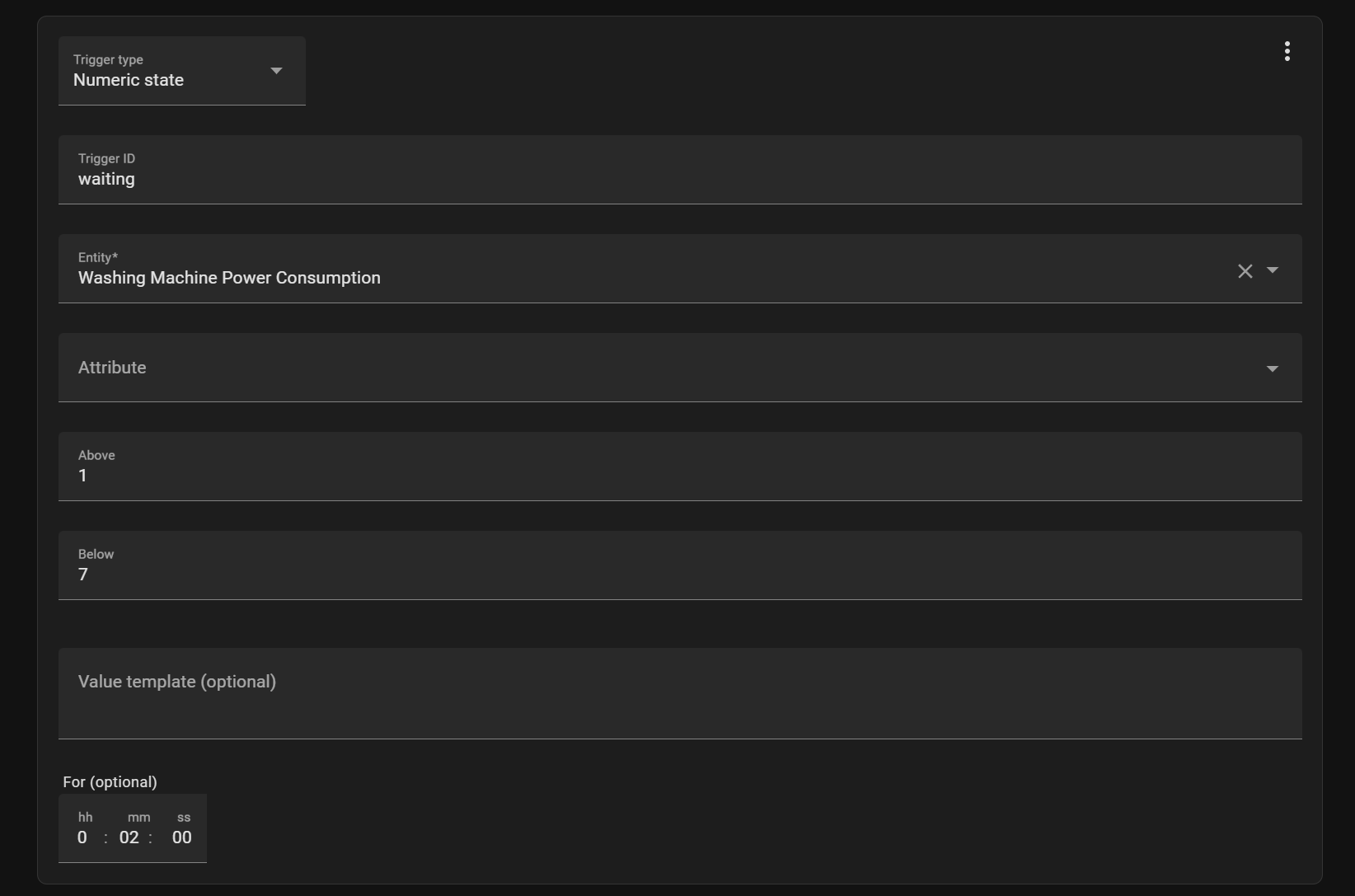The image features a structured layout with seven distinct rows, each bearing a title. The background of the image is black, with each row set against a lighter black square for contrast. At the bottom of these rows, there is a box that contains the number "4" followed by the word "optional" in parentheses.

In the forefront, white font text is prominently displayed. The text layout is as follows: 

- At the top, "HH" is positioned above "O", followed by a colon.
- Next to it, "MM" is placed above "A02", followed by another colon.
- Lastly, "SS" appears above "00".

Towards the top of the image, aligned to the left, the title "Trigger Type" is displayed, followed by the words "Numeric State" directly below it.

Subsequent details are aligned similarly:

- "Trigger ID" is listed with the word "Waiting" beneath it.
- "Entity" is specified, with "Washing Machine Power Consumption" written underneath.
- "Attribute" is stated, with "1" above and "7" below it.